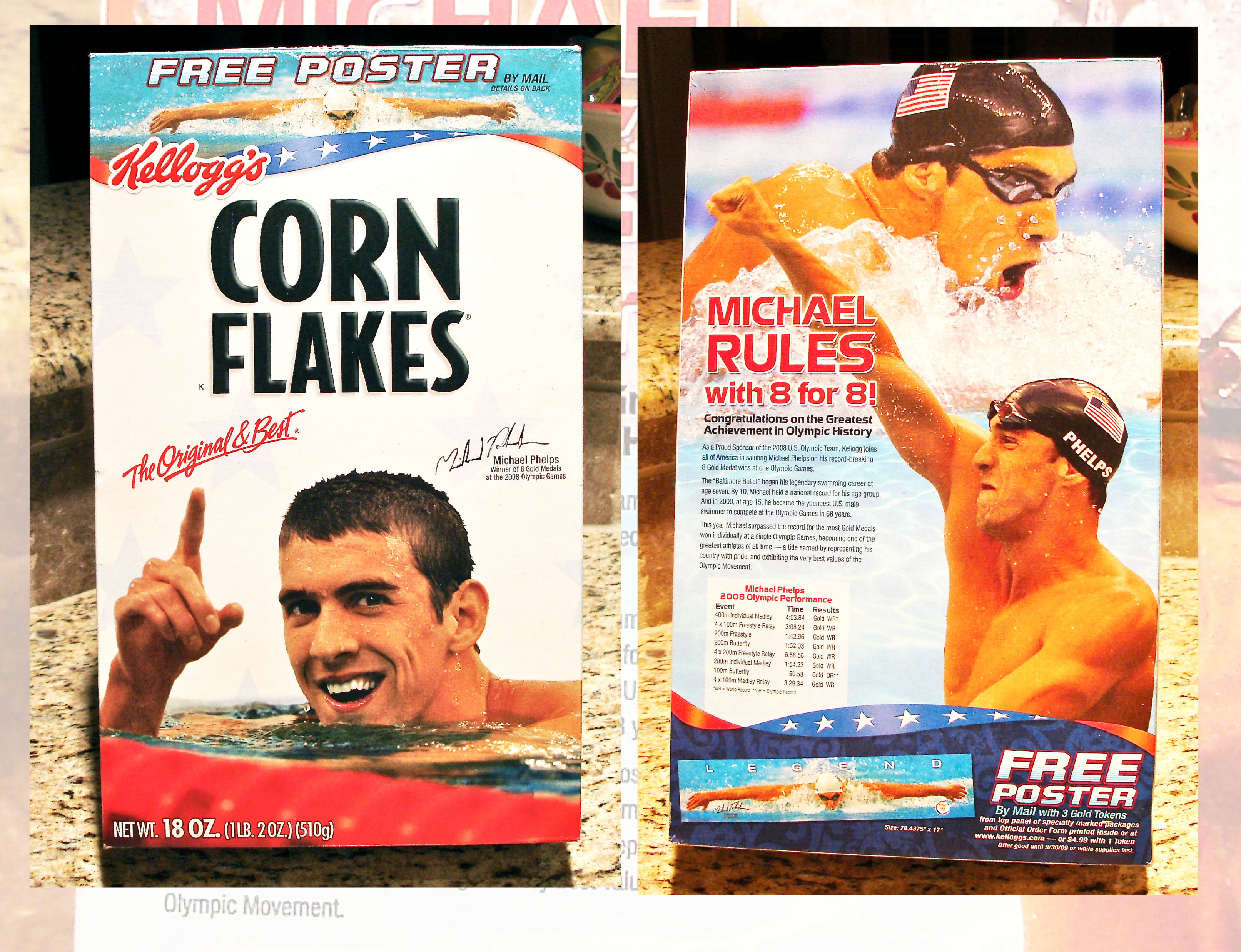This image showcases both the front and back of a Kellogg's Corn Flakes cereal box, prominently featuring Michael Phelps, the celebrated Olympic swimmer. On the left, the front of the box has a white background with bold black text reading "Corn Flakes," and beneath it, in red cursive, the phrase "The Original and Best." Towards the top, in thick white capital letters, the text reads "Free Poster by Mail, Details on the Back." At the center, there is a photograph of a young Michael Phelps, emerging from the water, smiling with short brown hair, and raising his right hand with the index finger pointing upward, signaling number one. His image aligns with the text "Michael Phelps, Winner of Eight Gold Medals at the 2008 Olympic Games," written in smaller text above his head, complete with his signature. At the very bottom left, the box indicates the net weight as "18 ounces, one pound, two ounces."

On the right side, the back of the box embellishes further on Phelps' achievements. It features two images of him: one mid-stroke in the water, wearing a black swim cap adorned with an American flag and goggles, and another showing him fist-pumping triumphantly. The text in the middle of this side of the box, written in red, reads "Michael Rules with Eight for Eight," celebrating his record-breaking performance. This side of the box appears to also contain detailed text probably comparing his Olympic times and achievements, alongside a likely nutritional chart. At the very bottom right, "Free Poster" is reiterated to draw attention to the promotion.